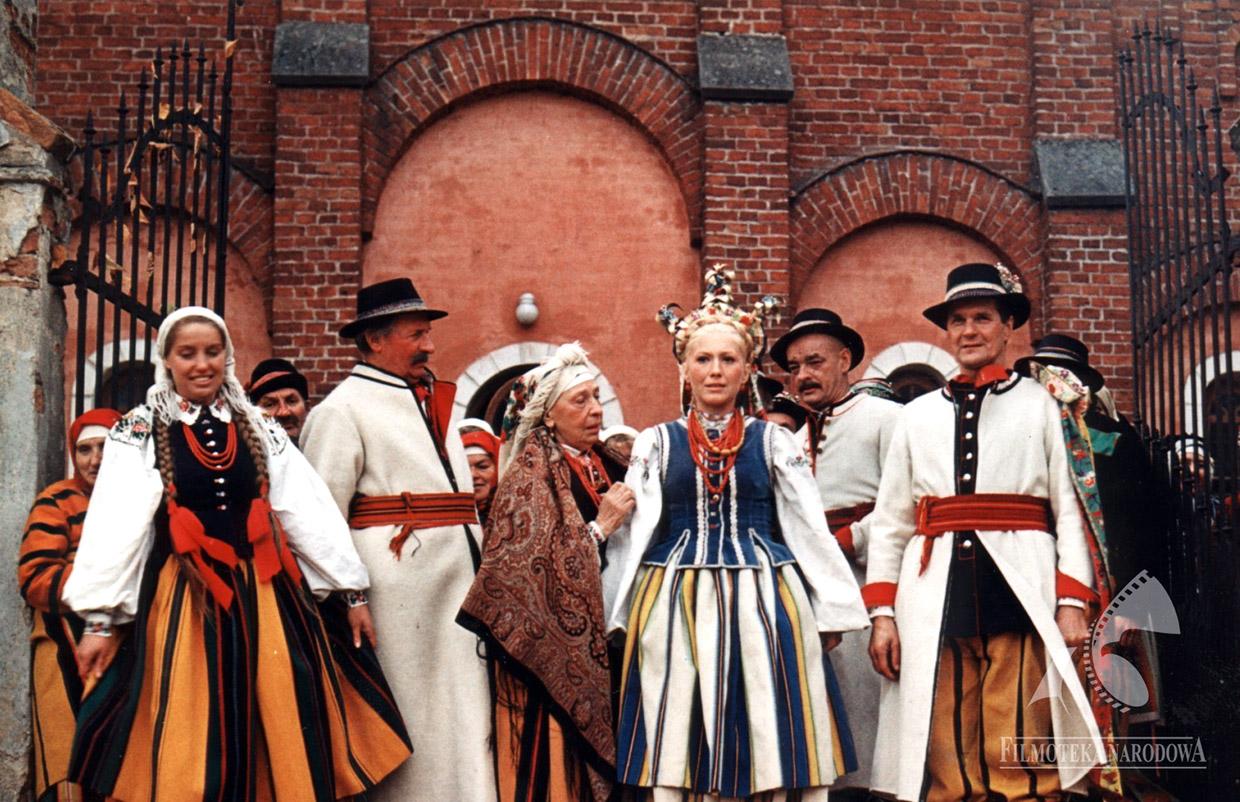This photo captures an outdoor cultural ceremony, potentially a celebration or wedding, set in front of a large brick church with prominent arches. A group of people is positioned between two black wrought iron gates. The watermark at the bottom reads "Filmotech Narodowa," indicating Polish origins and suggesting a cinematic context. The attendees are dressed in historical, traditional costumes. The women have their hair in pigtails and wear long, flowing skirts in various colors. Central among them is a possible queen or maiden, distinguished by a crown-like hair arrangement and a blue vest over a white blouse, with a striped blue, white, and golden-yellow dress. Another woman is seen in a burnt yellow and black striped dress, adorned with a black vest, red bows in her pigtails, and a white scarf over her head. The men wear long white coats with white buttons, black shirts with red bowties, and yellow-striped trousers. This detailed ensemble evokes a vivid image of a richly traditional and possibly cinematic scene.